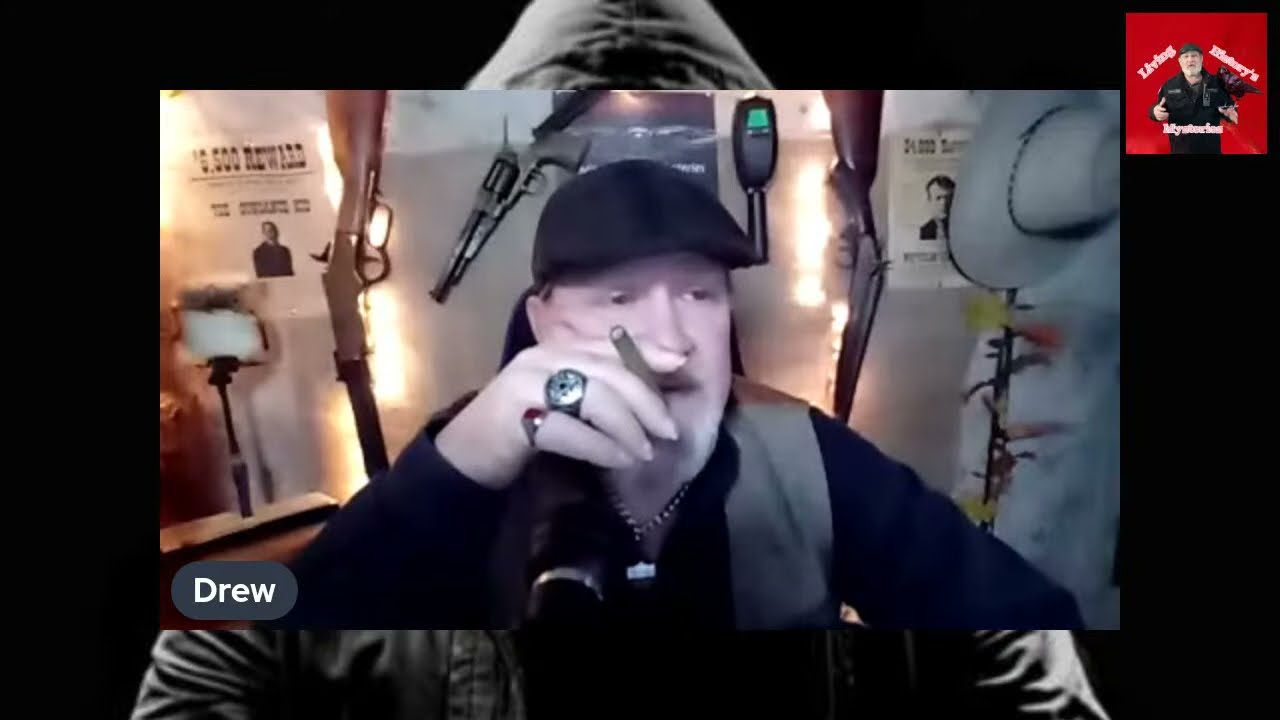The image is a layered composite featuring an individual named Drew prominently in the center. The primary focus is a photograph that is approximately 3 inches wide and 2 inches tall, depicting a Caucasian man seated behind a desk, possibly in an office or studio. He dons a black newsboy cap and a dark shirt under a light gray or tan vest. His left arm rests on a desk out of view, while his right hand, adorned with a large ring on the ring finger and a smaller ring with a red stone on the pinky, partially covers his face as he smokes a cigar. His chest is visible from about midway up, and he wears a noticeable necklace with beads and a pendant. A black microphone is in front of him. 

The background reveals a light-colored wall adorned with firearms, including rifles and handguns. Several posters are visible, one of which advertises a $5,500 reward, though it may actually state $6,500. A cowboy hat hangs near a walkie-talkie and some form of lighting. Over his left shoulder, another poster appears to be in a "wanted" format. In the lower left corner of the image, a grey oval displays the name "Drew" in white lettering. Opposite, in the top right corner of the larger image, there is a small red square showing Drew standing, with white text that includes the words "Living Histories" and an unclear second line, possibly "Mysteries."

The entire setup is framed by a larger black rectangle. At the very top, the upper edges of a gray hood are just visible, suggesting that the main photograph is placed on top of this image, where the lower part shows a portion of a gray jacket. In summary, the scene combines elements of an office or studio environment with a background decorated with memorabilia and personal items, highlighting Drew as the central figure in both seated and inset standing portraits.